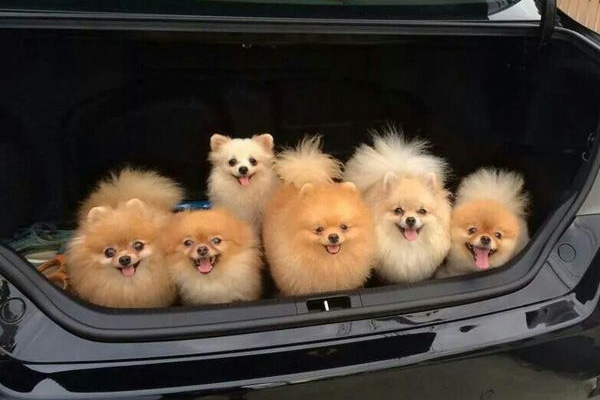In a horizontally aligned rectangular image, the back of a black vehicle is shown with its trunk open, revealing the interior. Inside the trunk are six fluffy Pomeranian dogs, all panting with their mouths open and tongues sticking out, giving the appearance of smiling. Their fur is predominantly brown and incredibly puffy, with spiky tufts making them look larger and more adorable. The dogs have large brown eyes and tiny ears mostly covered by their luxuriant coats. The vehicle is parked next to a brown wall with a line pattern, and the ground below appears dark gray or black. The scene is brightly lit, suggesting it is taken during the daytime. The backdrop of the image remains focused on these cheerful, photogenic pups, all captivated and looking directly at the camera.